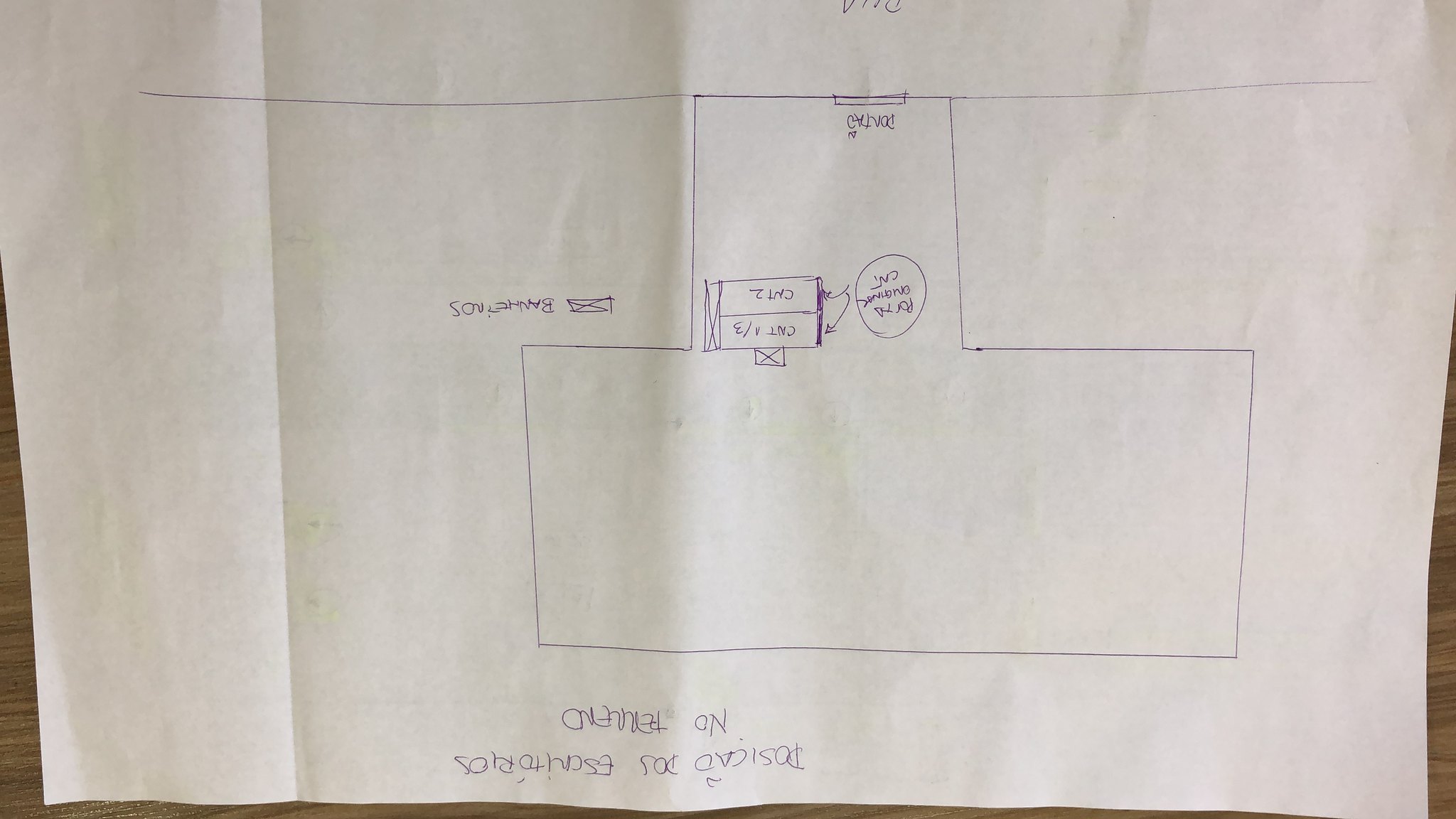This image features a hand-drawn sketch of a simplistic floor plan, rendered with thin lines and predominantly right angles. The sketch is oriented upside down, as indicated by the non-English letters and numbers. The layout resembles a bulky, inverted letter "T," with the crossbar of the "T" extending further to the right than to the left. Within the main vertical section of the "T," two small rectangles are drawn, each containing some non-English text. Outside the "T" structure, a box marked with an "X" can be seen, also containing some writing that is illegible. The sketch is drawn on white paper, which shows a visible crease suggesting it has been folded at some point.